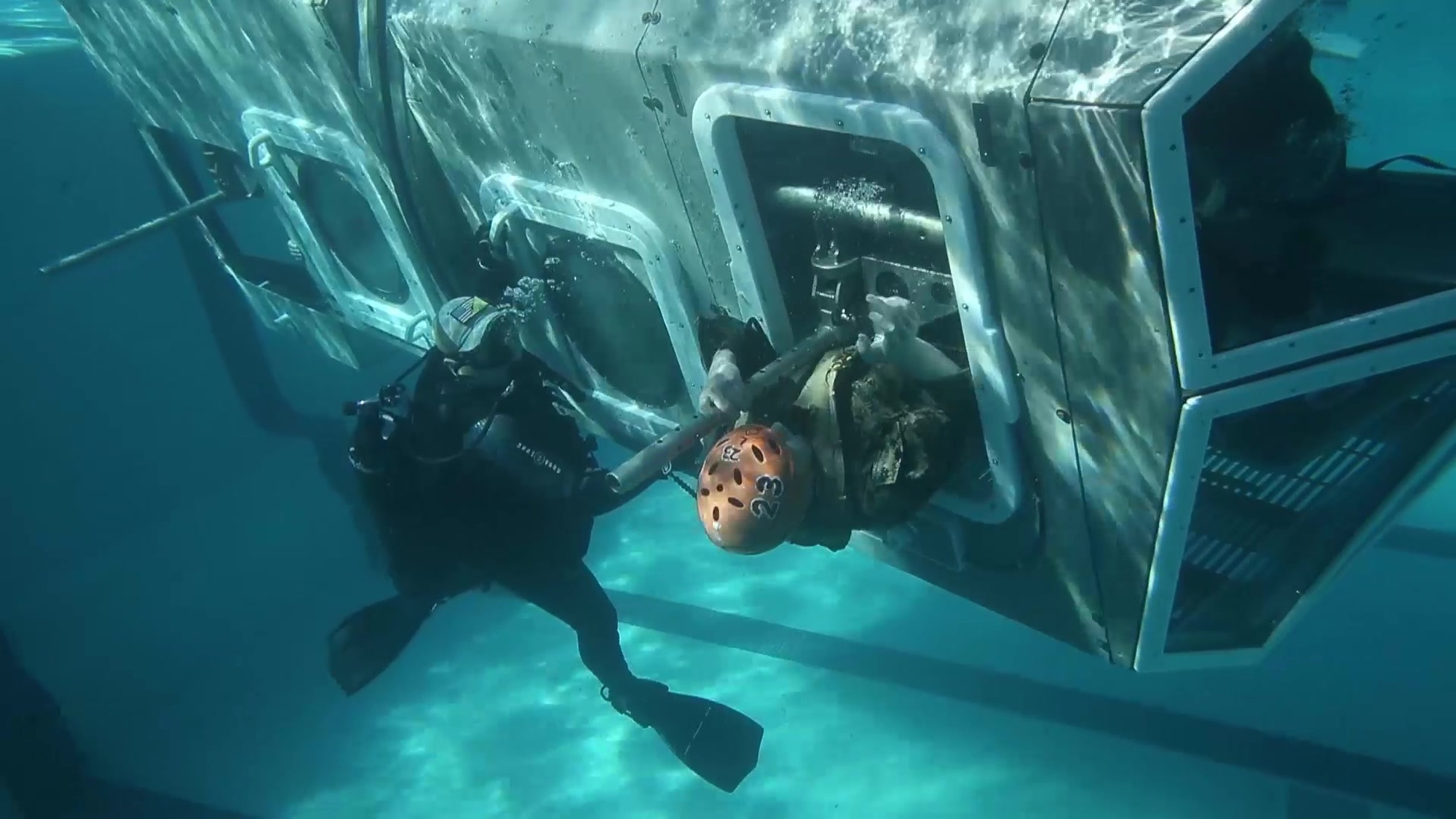This underwater photograph, taken in a blue swimming pool, features two men involved in a military training exercise. The central figure is emerging from a submerged, armored vehicle simulator resembling a Dilbert Dunker. He wears a green camouflage uniform, white gloves, and an orange helmet marked with the number 23. The man appears to be holding a pipe as he pulls himself out of the vehicle. His right hand is in a gesture that looks like he's flipping the bird. Beside him, another man in snorkeling gear, equipped with a mouthpiece rebreather, observes closely. This assistant wears a baseball cap adorned with an American flag and camouflage design. The pool background includes lines running along the sidewall and floor, adding depth to the scene.